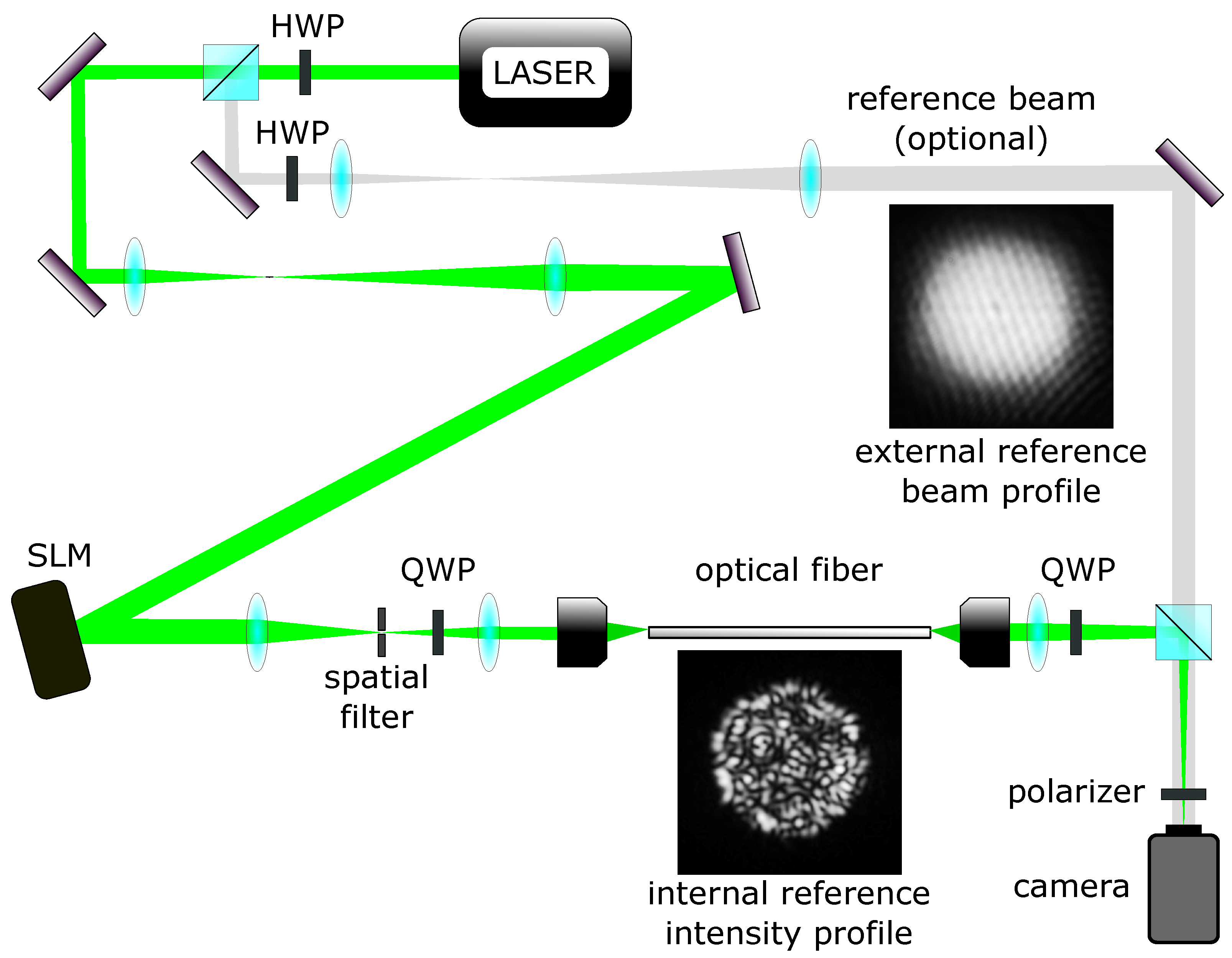This image is a detailed scientific diagram of a laser and optical-driven model. At the top, a laser emits a green line representing its path, which is labeled HWP (Half-Wave Plate). The diagram features a complex zigzag pathway with various labels and symbols indicating the laser's interaction with different optical components. Small cylinders mark each sharp turn in the pathway, accompanied by translucent aqua blue ellipses that likely represent lenses.

Highlighted in the diagram are several key abbreviations and components. The laser beam first encounters a Half-Wave Plate (HWP) before proceeding through the path marked by metallic-looking cylinders and lenses. The path continues to an SLM (Spatial Light Modulator), depicted as a rounded black rectangle, and follows through several more ellipses to a QWP (Quarter-Wave Plate), down to a spatial filter, and ultimately connects to an optical fiber—a long white tube with black caps on either end.

In the bottom right, a camera icon is shown with a polarizer above it. The diagram also includes labels for an internal reference intensity profile, which is represented by an image of a flash below the optical fiber. Additionally, an optional reference beam path is marked in the upper left, leading to another HWP and an external reference beam profile.

The color scheme consists of black, white, light blue, steel gray, and green, adding to the intricate and somewhat complicated appearance of this scientific representation of the laser's pathway through various optical elements.